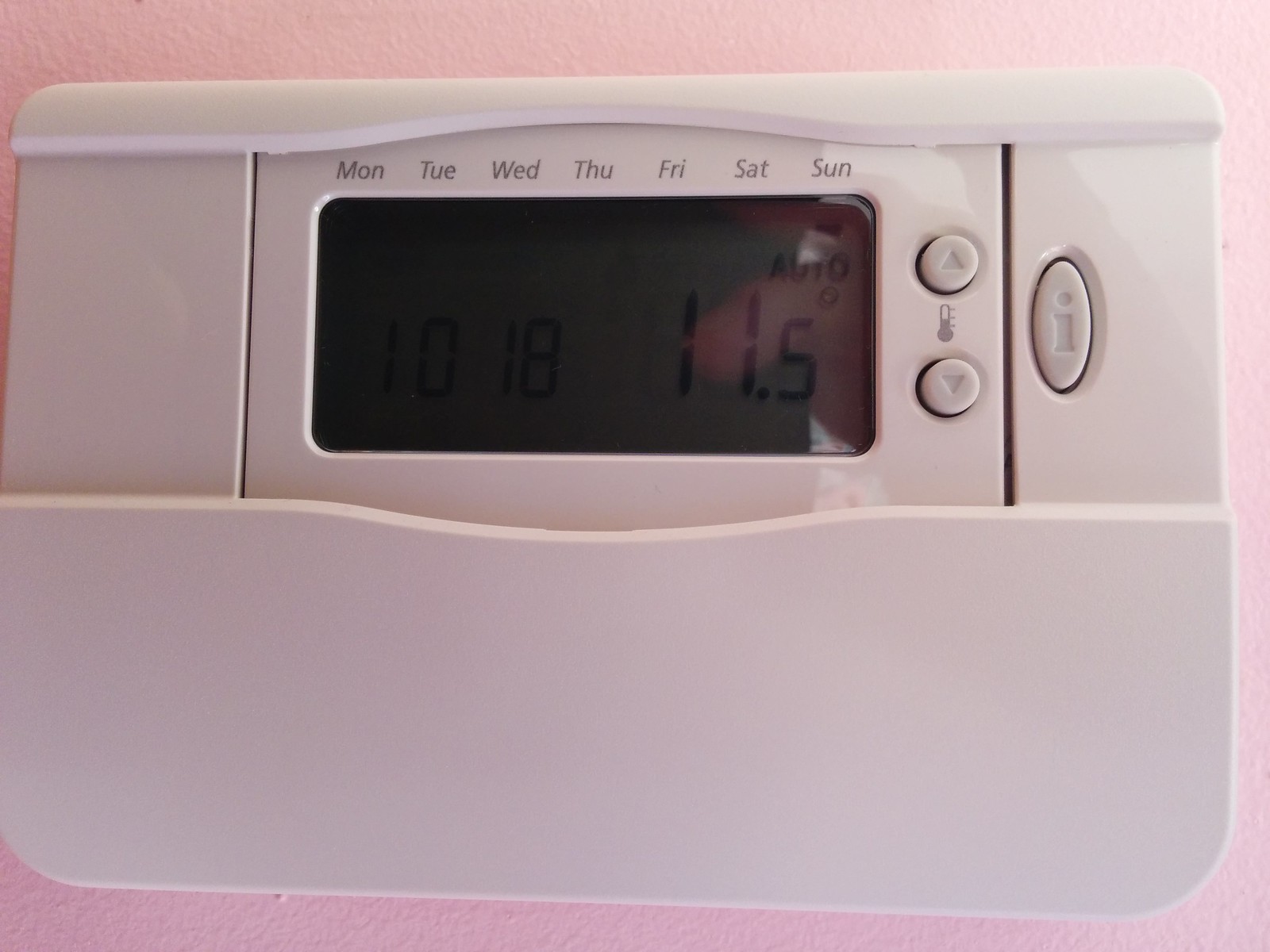This close-up photograph captures a white thermostat prominently displayed on a pink wall, filling the majority of the frame. The thermostat features a distinctive lid design, with a small horizontal section at the top that curves upward at the center, mirrored by a wider bottom section with the same vertical curvature. The centerpiece of the thermostat elegantly displays the days of the week, Monday to Sunday, each day beginning with a capital letter.

Beneath the days of the week, a digital window display, though dark in the photograph, reveals essential information, likely including the time and temperature. Within this display, the number "11.5" is faintly visible, and the setting is noted as "auto." Flanking the display on the right are two vertically aligned circular buttons, each adorned with a triangle pointing either upward or downward, allowing for temperature adjustments. Positioned between these buttons is a small thermometer icon, indicating their function.

Adjacent to this setup is an oval button marked with the letter "I," suggesting an additional control feature, though its exact purpose remains unspecified. To the left of the display, a blank section forms its own distinct area, adding to the thermostat's sleek and organized design.